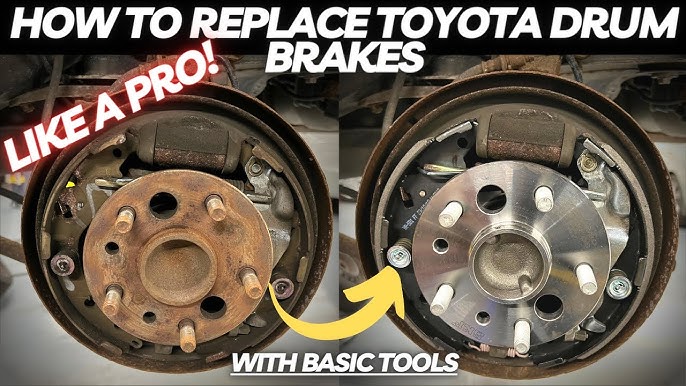The image is a detailed thumbnail for a YouTube video titled "How to Replace Toyota Drum Brakes." It features large white capital text at the top with the video's title, and at the bottom, also in white underlined text, it reads "With Basic Tools." Diagonally across the top left, "LIKE A PRO!" is emphasized in white text with a red fuzzy background. The central image is split in half, showing a comparison between an old, rusty Toyota drum brake on the left and a new, shiny silver drum brake on the right. A yellow arrow swoops from the left side to the right, highlighting the transformation process. The visual contrast between the two sides underscores the improvement achieved by replacing the drum brakes using basic tools, as the video promises.